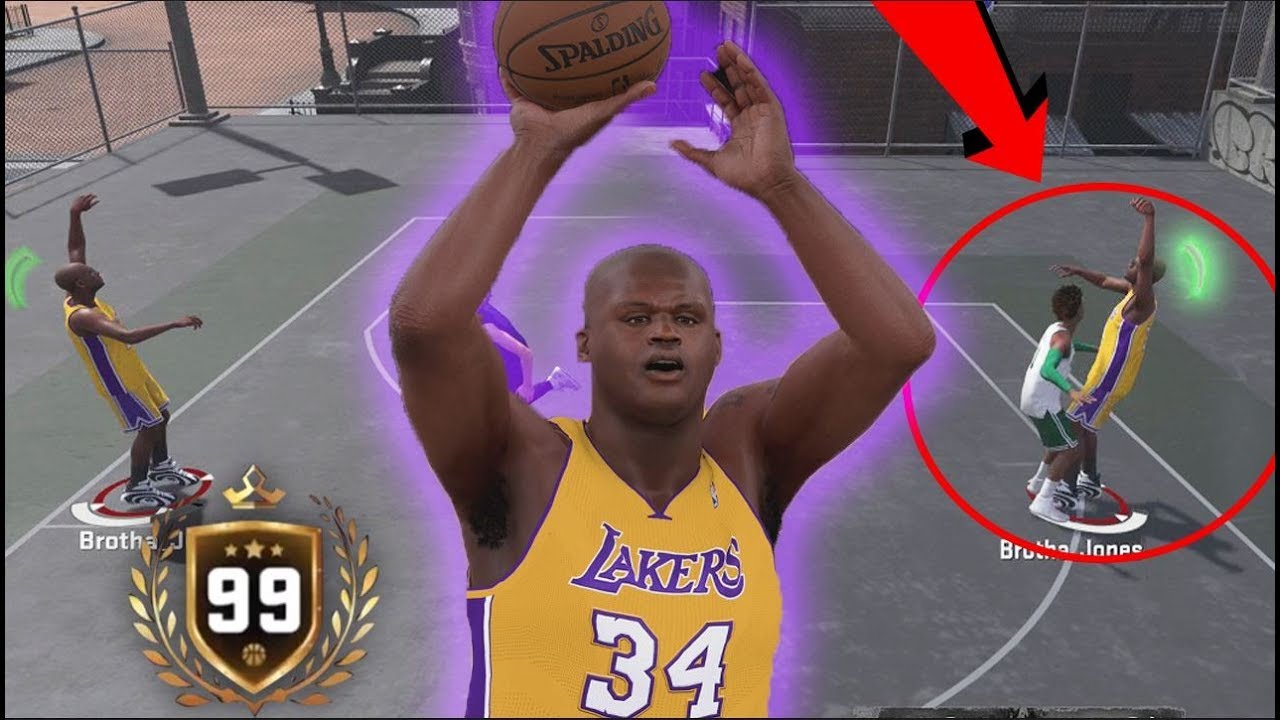In this detailed image, which seems to be derived from a video game or animation, the scene is set on a gritty, urban street-style basketball court complete with a cement surface and chain-link fences typical of a neighborhood park. Dominating the center of the image is a somewhat poorly rendered computer-generated figure of Shaquille O'Neal, identifiable by his Lakers jersey emblazoned with the number 34. He's captured holding a basketball, embodying his iconic stance. To the left of Shaquille O'Neal is another Lakers player, who might be a possible duplicate of O'Neal. On the right side, the scene depicts a close interaction between another Lakers player and an opponent donning a white tank top and green shorts, adding a dynamic element to the gameplay. At the bottom of the image, a ranking emblem prominently displays the number 99, suggesting a high rating or level within the context of the game.